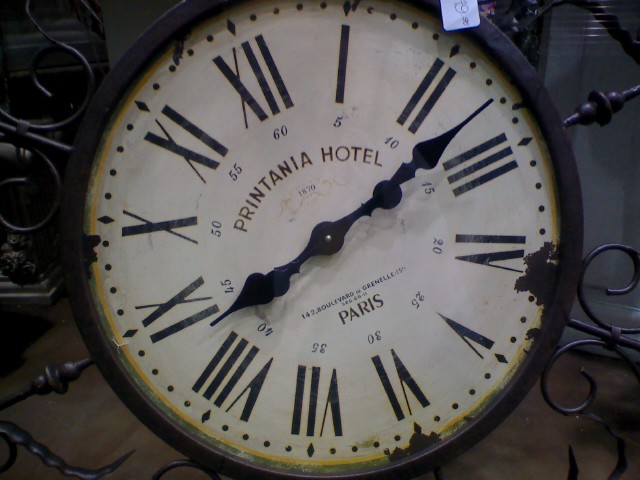This image showcases a vintage, ornate clock with a black metal ring encircling its off-white face, which exudes an antique charm with its chipped and slightly rusted surface. The clock is adorned with black Roman numerals and features distinctive hands resembling spade symbols from a deck of cards. Prominently displayed on the clock's face are the words "Printania Hotel," elegantly curved in the center, and beneath it, "Boulevard de Grenelle, Paris" is inscribed, denoting its origin. The clock is mounted against a backdrop of intricate black wrought iron, reminiscent of Victorian-era artistry, with elaborate curls and straight bars affixed to the perimeter, adding to its timeless appeal. A subtle yellow ring accentuates the exterior edge of the clock face, enhancing its historic aesthetic.